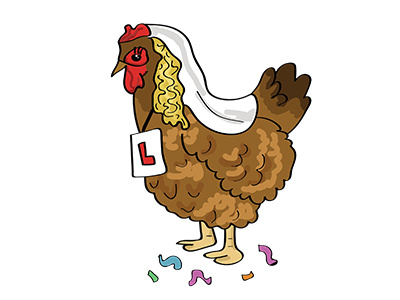The image is a detailed cartoon-style rendering of a rooster. The rooster is predominantly brown with various shades adding depth to its plumage, including darker brown details on its tail. It has distinctive red features such as a comb on its head and a waddle. The eyes are black in the center, surrounded by red accents. Notably, the rooster is wearing a white wedding veil along with blonde hair, suggesting a quirky character about to get married. Around its neck, there is a white rectangular piece of paper with a red letter "L" on it, like a makeshift necklace. Confetti in colors such as purple, orange, blue, and green is scattered on the ground around its feet. The overall scene is set against a plain white background, placing full emphasis on the amusingly dressed rooster and the festive confetti surrounding it.